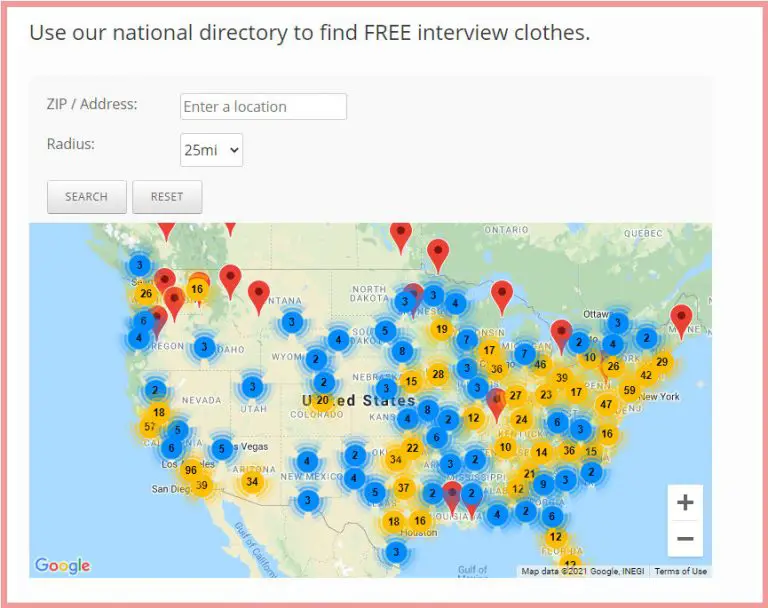The image displays a section of a website with an interactive map focused on the United States. The map shows outlines of U.S. states, with parts of Ontario and Quebec from Canada visible to the north, and a portion of Mexico visible to the south. The map lacks detailed information on each state but provides a general overview.

On the right side of the map, there are plus and minus buttons for zooming in and out. The bottom left corner features a "Google" watermark, indicating that the map is powered by Google Maps. Coastal bodies of water are also visible along the edges of the map.

Numerous location icons are scattered across the map, predominantly concentrated on the East Coast around the New York area. These icons are colored yellow and blue. Additionally, some locations are marked with traditional red balloon icons.

Above the map, a header reads "Use our national directory to find a free interview close." Below this header, there is a form field with prompts for entering a zip code or address, along with a drop-down menu to select a search radius, defaulting to 25 miles. Two buttons—one for searching and one for resetting the map—are also present over the map.